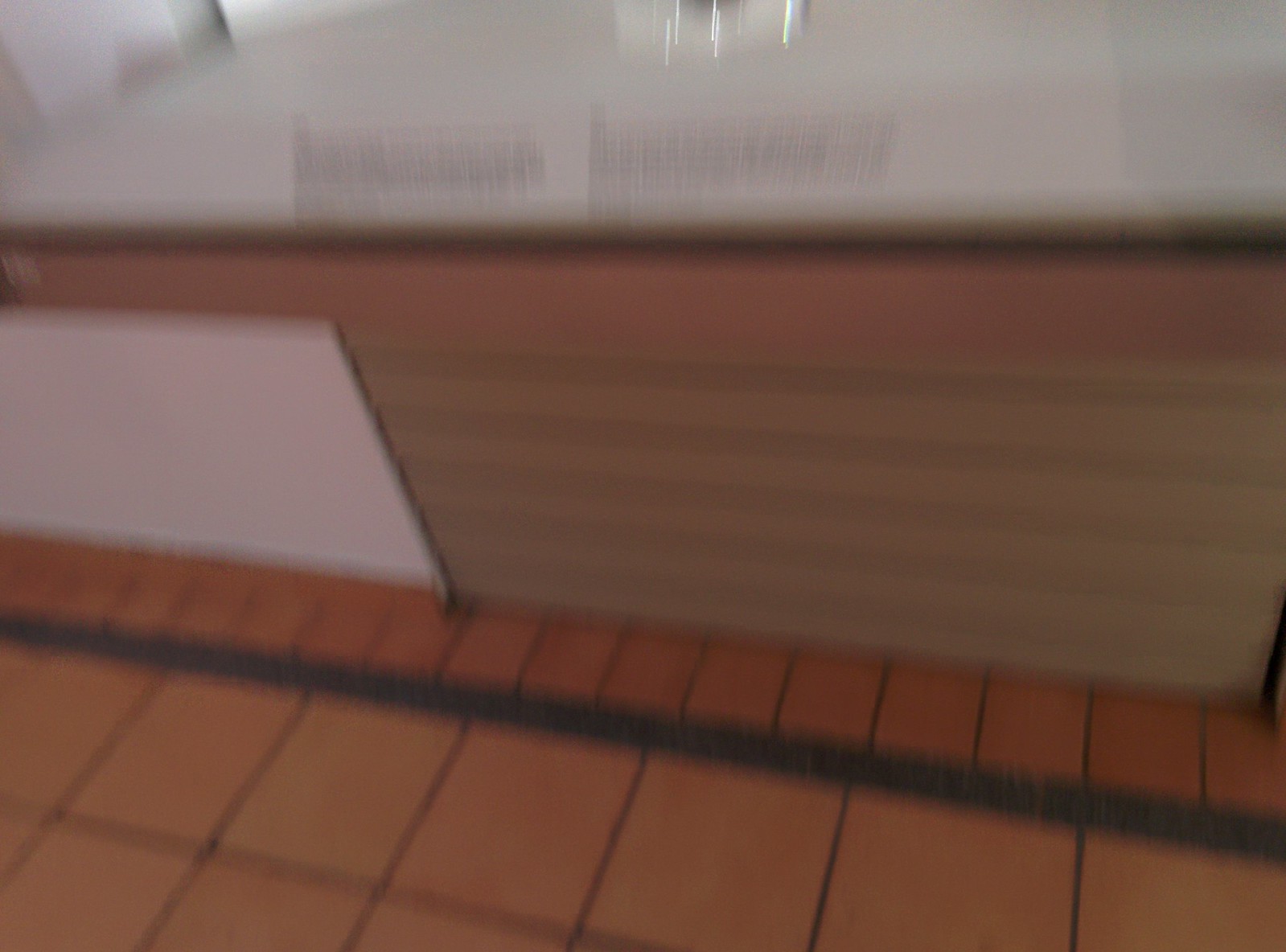The image is a close-up, slightly blurry photo, likely taken from a first-person perspective and possibly while in motion. The lower part of the image, which is more in focus, shows a floor with dark orange square tiles bordered by lines of black or dark graphite. Near the middle of the image, there is a transitional strip featuring smaller square tiles, which are about one-third to two-thirds the size of the larger ones. These smaller tiles are set against a white wall, which is adorned with what looks like light brown shutters. The top half of the image is out of focus, revealing a possible counter displaying indistinct black letters on a white background, suggesting signs or a menu. There is a shimmer of light or a reflection on the counter, indicating a polished surface. Overall, the scene seems to be inside a store or a café, with ceiling lights faintly reflecting on the countertop.